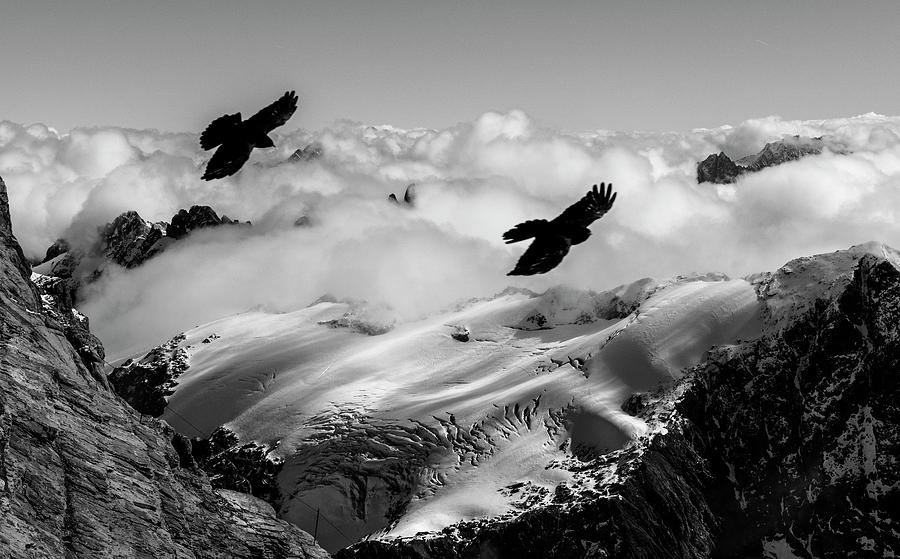This striking black and white photograph, reminiscent of Ansel Adams' work due to its high-contrast values, captures a dramatic mountainous landscape cloaked in thick, puffy clouds. Taken from a high vantage point, the image showcases the rugged terrain with a snow-covered slope in the foreground and jagged, rocky peaks flanking the scene on both sides. The right peak sports a dusting of snow, while the left remains bare and rough-textured. 

Amidst this natural grandeur, two small, dark-colored birds, possibly hawks, are gracefully soaring with their wings outstretched. Positioned near the center of the image, the bird on the left flies higher as they glides over the mountain range, seemingly riding thermal updrafts. Their elegant flight occurs against a backdrop of thick clouds that obscure the peaks in the distance, leaving only their tips visible. The sky, emerging clear above the clouds, hints at the late evening sunlight filtering through from the right, casting subtle highlights on the scene below. This photograph beautifully encapsulates the serene yet powerful essence of mountain wilderness and avian flight.